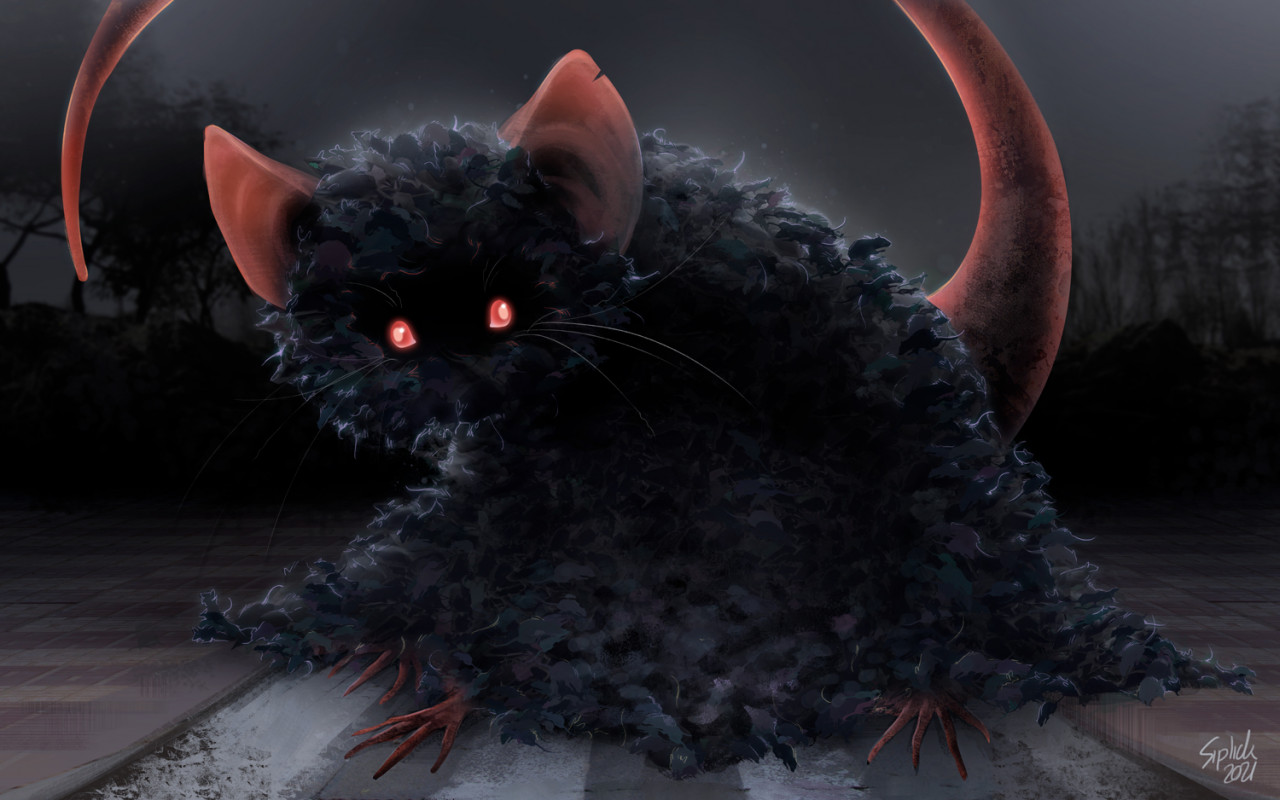The image showcases a computer-generated or painted fantasy depiction of a surreal, cartoonish black rat with horror elements. The creature, composed of clumps of dark hair resembling other rats or possibly black yarn, has piercing, glowing red eyes and large, pointy, light-red ears. A long, pink, rat-like tail curls above its body, adding to its eerie appearance. The rat is positioned on a brick or wooden surface, with its spindly, stick-like legs and pointy, clawed toes visible—three feet can be distinctly seen. The background features a dark sky and the silhouettes of trees on both sides, creating a foreboding atmosphere. In the right corner, there is a name with the date 2021, indicating the artwork's creation. The rat's glowing eyes appear to follow the viewer, enhancing the unsettling, fantastical nature of the image.